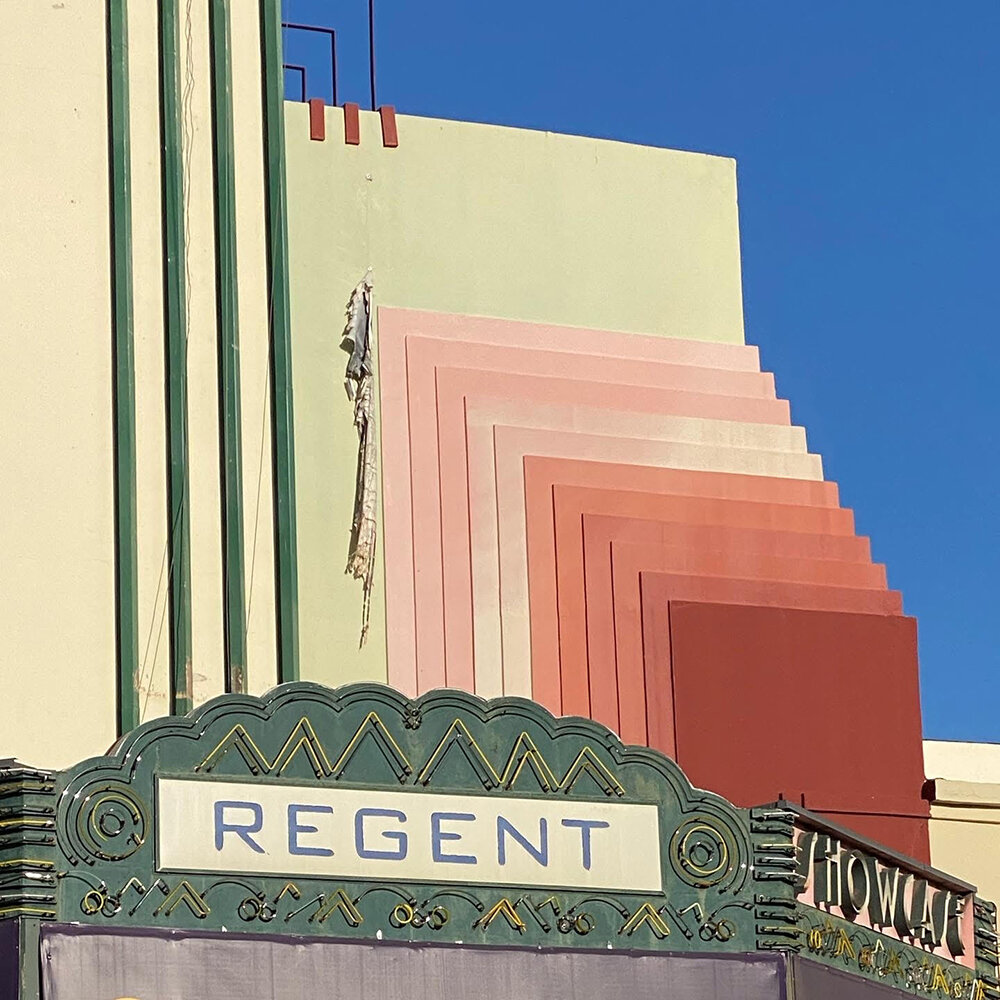The image depicts the exterior of an elaborate building that resembles an old theater, prominently featuring a long white rectangular sign with blue letters that spell "Regent". To the right of this sign, in cast letters, it says "Showcase". Above the signage, the building's facade is adorned with a striking design composed of cascading squares, each layer slightly larger as they ascend. Starting with a blood-red square at the bottom, the squares lighten progressively through shades of terracotta and pink, creating a textured and layered appearance until they reach a light pink at the top. The colorful squares are set against a greenish backboard on the left and a blue background on the right, creating a visually captivating, unconventional design. The sky in the top right corner of the image is a medium blue, clear, and free of clouds. Additionally, a tattered, old vinyl sign hangs precariously above the squares, adding a touch of historical wear to the surreal, almost art-like facade.